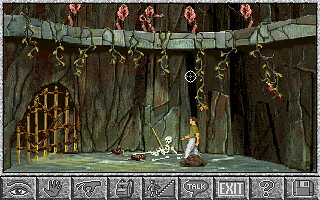In this color image, likely a scene from a computer game, the details are quite small and somewhat indistinct. At the bottom of the image, there is a grey, rock-like line adorned with approximately ten square-shaped symbols, though they are hard to decipher. Among these symbols is an exit icon, positioned centrally among the game's control indicators. 

A prominent green sign is visible, adding a splash of color to the scene. On the left side, an archway features yellow bars extending vertically, enhancing the impression of a cave setting. This cave-like atmosphere is further accentuated by yellow tendrils or light strands that drape over the ceiling, descending from a grey, blocky line running horizontally across the image.

In the center of the scene, a small character, dressed in a green top and white trousers, stands out. Beside this character, there appears to be a smaller figure, possibly a dog. Pink objects are scattered across the top of the image, though their exact nature is unclear. Overall, the image conveys a mysterious, cave-like environment with elements of a computer game interface.